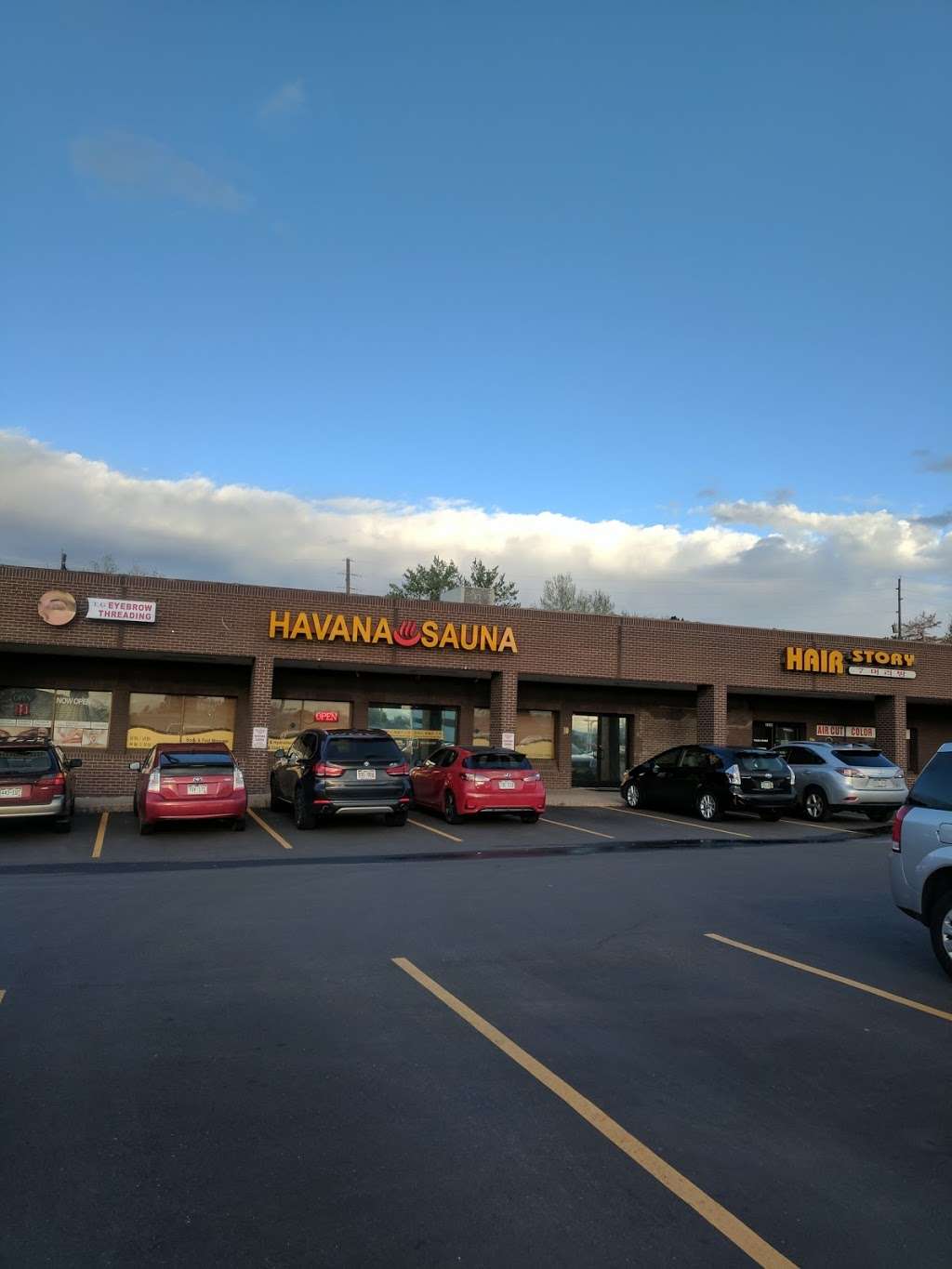The image depicts a strip mall with three visible stores: Eyebrow Threading, Havana Sauna, and Hair Story, with their signs displayed prominently above. The scene is set during daylight, with a blue sky and a layer of white and gray clouds near the horizon. In the parking lot, seven vehicles are parked: two black, two silver, two red, and one burgundy. Six of these vehicles are positioned in the front row facing the storefronts, while the seventh, a silver car, is located closer to the foreground, showing its side. Yellow parking lines on the dark gray asphalt are clearly marked, indicating a well-maintained parking lot. Signs such as "Now Open," "Open," and "Haircut and Color" are visible, and there's some water trailing down the lot. The photo captures low cloud tops and hints of trees above the building.